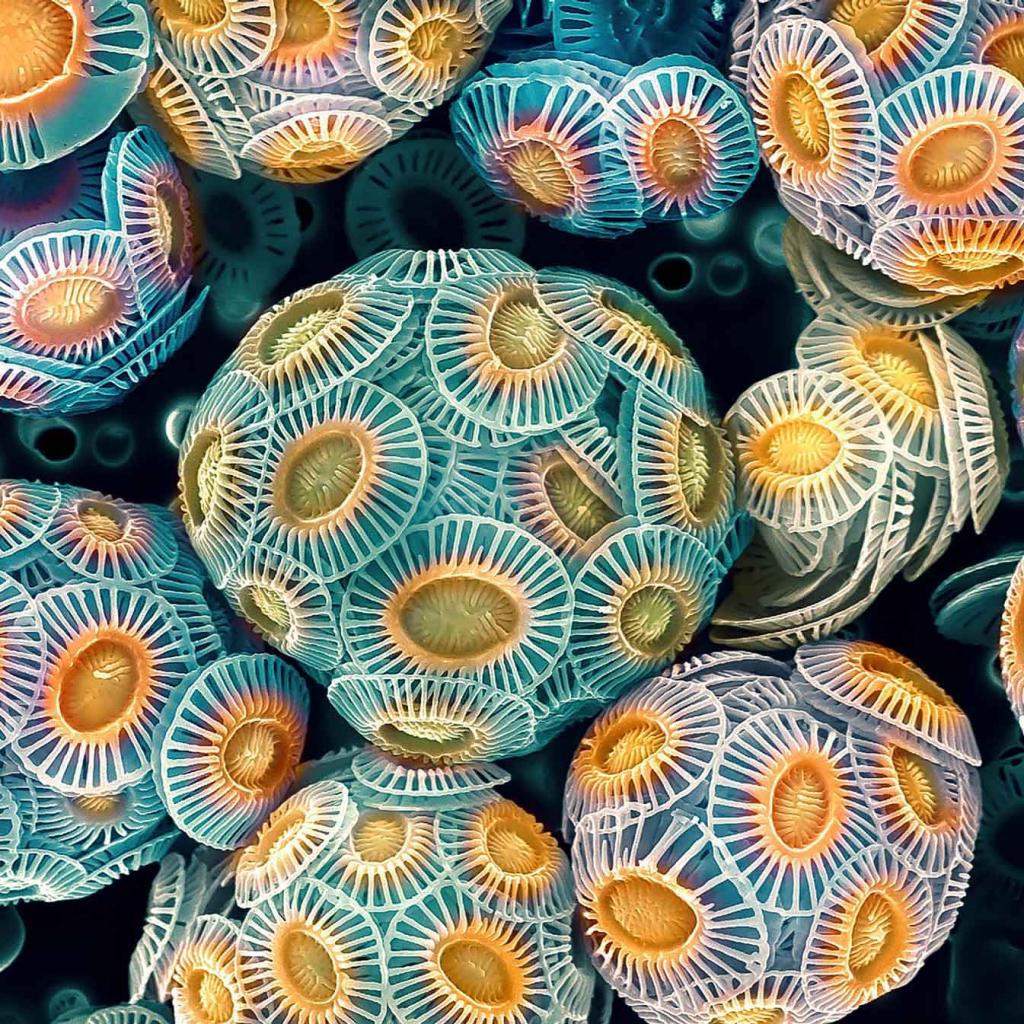This image appears to be an abstract, possibly AI-generated, highly detailed and textured 3D artwork or high-resolution photograph. The predominant background is a gradient transitioning from light to darker shades of blue, verging on black. At the center of attention are several spherical formations—around eight in total—each composed of multiple smaller, intricate elements that resemble sand dollars or perhaps microscopic organisms like plankton or bacteria. 

These sand dollar-like elements have a striking light blue coloration with vibrant yellow central circles, and they are clustered together to form larger spherical structures. The spheres feature additional characteristics such as white rings and lines radiating from their centers, adding to the overall complexity and texture. The spheres, some of which appear fragmented while others remain whole, float against the atmospheric backdrop, with the entire composition displaying a range of vivid colors including yellow, orange, blue, and white. The image contains no text or discernible animals or mechanical structures, leaving its exact nature open to interpretation.